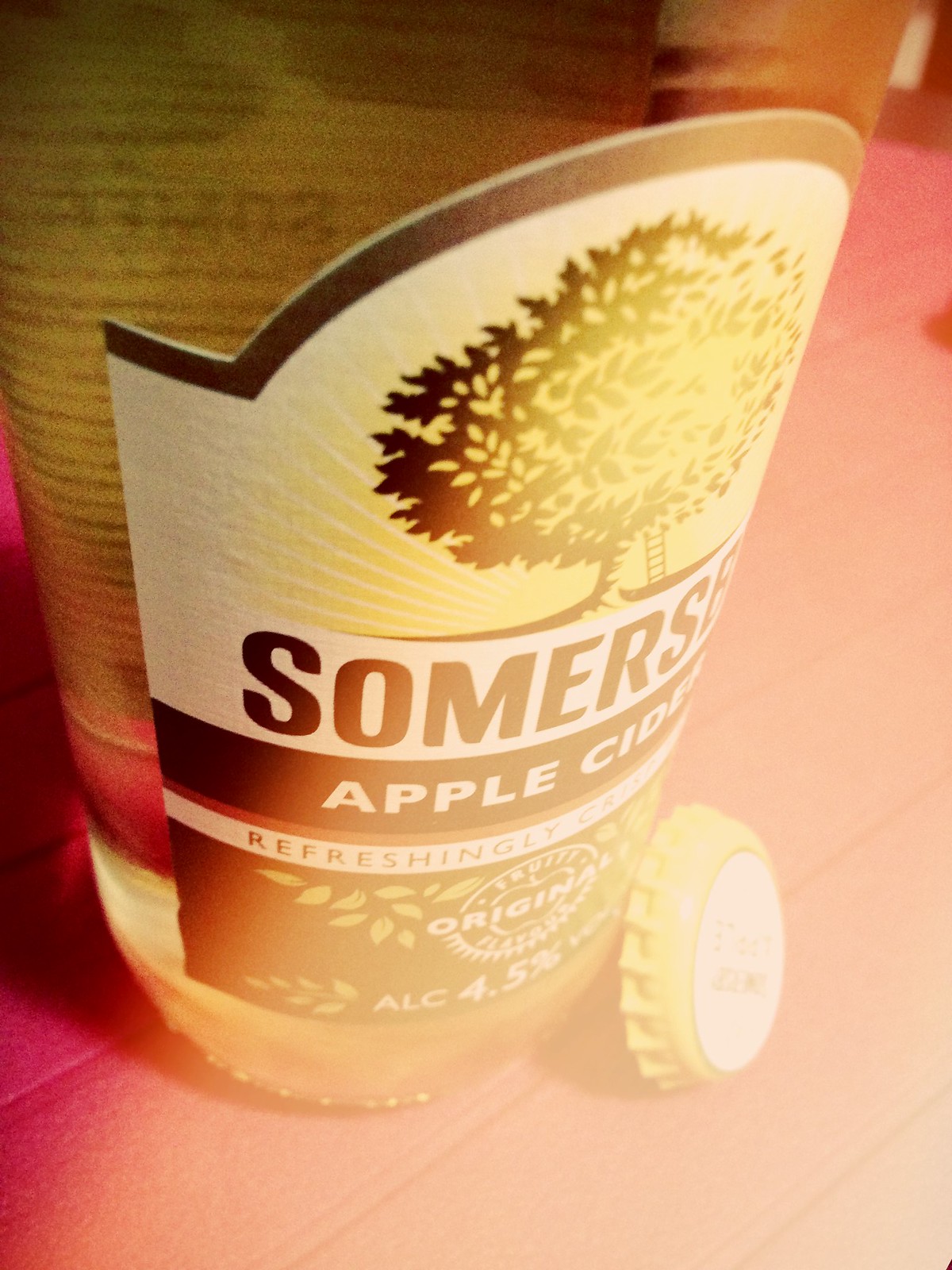This close-up photo captures a semi-clear, slightly angled bottle of Somerset Apple Cider, showcasing its detailed label. The photo, taken from a slight top-down perspective, makes the top of the bottle appear larger than the bottom. The label features an arch with an illustrated tree at the top, which has a thin trunk, a large bushy canopy, and a small ladder on the right. The tree has sunburst designs radiating from behind it. 

Above the tree, the brand name "Somerset" is partially visible. Below the tree, the large black text reads "Somerset Apple Cider" followed by a smaller, less legible text, "Refreshingly," suggesting a continuation that wraps around the bottle. Further down, in smaller print, it reads "original" surrounded by a leafy design, and below this is another badge or circle with an apple in the center. Just beneath this, the text indicates an alcohol content of 4.5%.

The bottle cap rests against the bottle, and the entire image has been heavily edited with an Instagram filter, creating a gradient from a bright, high-contrast top to a washed-out, peachy bottom, adding a unique visual effect to the photo.